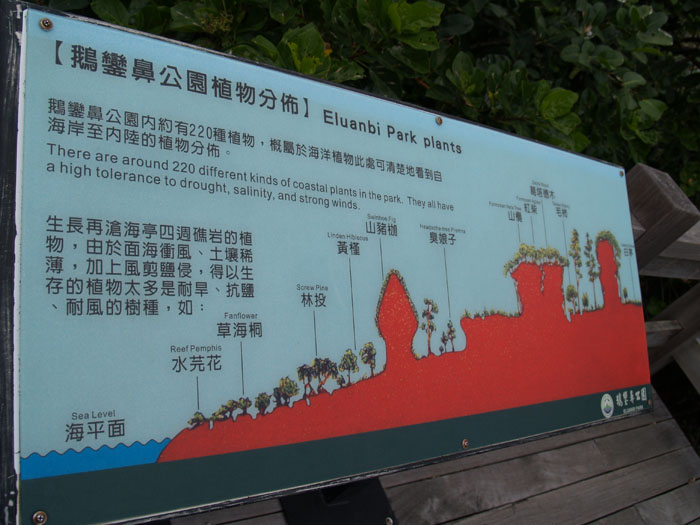The image depicts an informational placard for L1B Park, detailing the various plant species found at different elevations within the park. The placard is rectangular, white, and predominantly written in Chinese, making it difficult to decipher for non-Chinese speakers. It showcases a gradient elevation from sea level upwards, highlighting various coastal plants that thrive in these conditions. The bottom part of the placard represents the ocean or water, with a red silhouette illustrating the land of the park as it rises. Each plant is meticulously drawn and labeled, starting from sea level with reef plants and moving upward to feature species like pemphis, fanflower, screw pine, linden, hibiscus, and others that become harder to identify due to the distance from the camera and language barriers. Notably, the red land is outlined in contrast to the blue sky at the top. The placard explains that the park hosts around 220 kinds of coastal plants, all with high tolerance to drought, salinity, and strong winds, each identified with lines connecting to their respective illustrations.